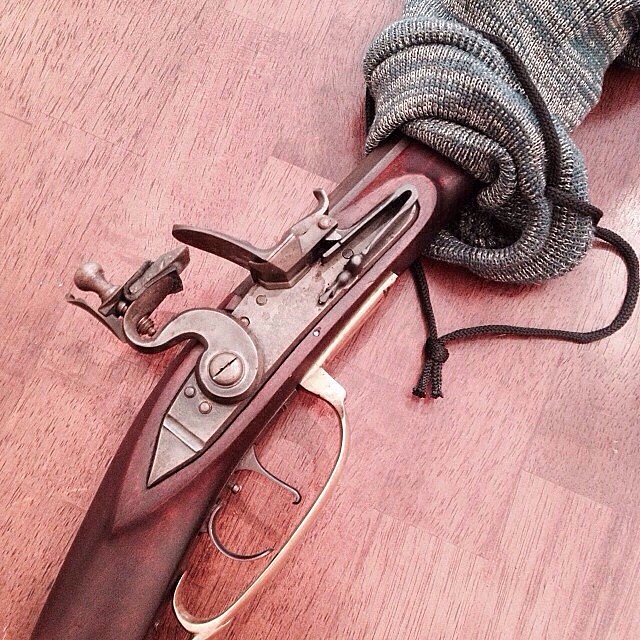This image captures a close-up view of an antique, vintage Western firearm, likely dating back to the early 1800s. The gun is positioned at a 45-degree angle on a wooden floor composed of reddish strips, enhancing the aesthetic and historical charm. The firearm itself features a beautifully patinated red mahogany wooden body with intricate metal fittings, including a well-preserved trigger mechanism. Notably, the muzzle is protected by a tightly woven, grayish yarn fabric cover secured with a brown drawstring, suggesting efforts for preservation. The overall design hints at a musket or similar historical weapon, emphasizing its age and bygone-era craftsmanship.